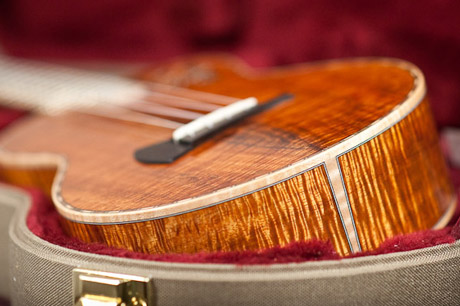This vivid close-up photograph captures the lower portion of a wooden string instrument, possibly a guitar or ukulele, resting in an open case. The instrument is carved from dark mahogany wood with lighter textured streaks. Its white strings are anchored by a black bridge and a white saddle. The shot is tightly framed, with most of the instrument appearing blurred, except for the clearly visible parts near the bottom. The instrument is nestled into the case, which has a rich, fuzzy red interior. A gold metal clasp is visible at the bottom of the case, and the exterior of the case appears to be woven tan fabric. The background behind the instrument is predominantly red with black accents, providing a striking contrast to the darker tones of the instrument and the texture of the case.